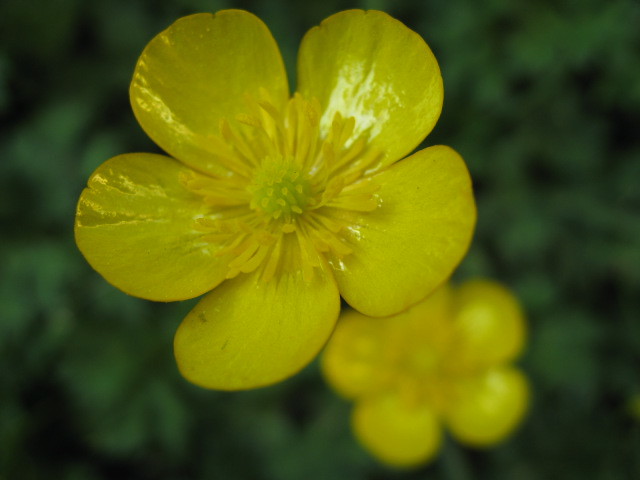This image showcases an up-close view of a vibrant yellow buttercup flower with five rounded, slightly shiny petals. The flower's center is green, featuring a circular arrangement with yellow dots and longer yellow projections, indicative of stamen and pollen structures. Behind the prominent flower, a smaller, slightly obscured yellow flower can be seen, also with five petals. The background comprises blurred green leaves, adding a lush, verdant backdrop that suggests the presence of grass or possibly a garden or greenhouse setting, enhancing the botanical richness of the scene.